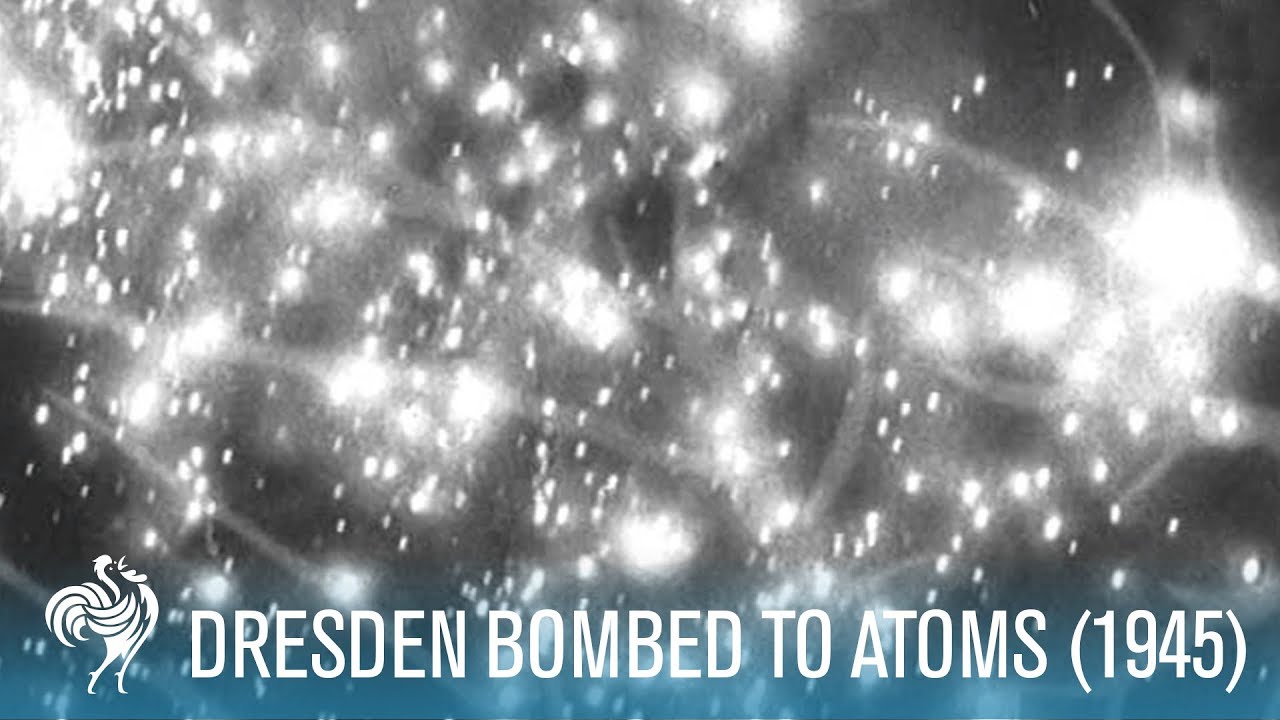This black and white image is an abstract depiction of what appears to be a night sky filled with numerous stars, rendered with a blurred effect that obscures precise details. The stars are shown as bright white lights against the dark sky, with some areas displaying white, faded streaks and smoky protrusions emanating from the larger white spots. The ambiguity of the scene contributes to an overall sense of mystery. Along the bottom of the image, a smaller section stands out due to a logo depicting either a dancing chicken or a lady, placed beside a cockerel facing right and crowing upwards. Accompanying this logo is the text "Dresden Bombed to Atoms" followed by the date "1945" in parentheses, all in white font. This text suggests the image might represent or be connected to the bombing of Dresden during World War II.